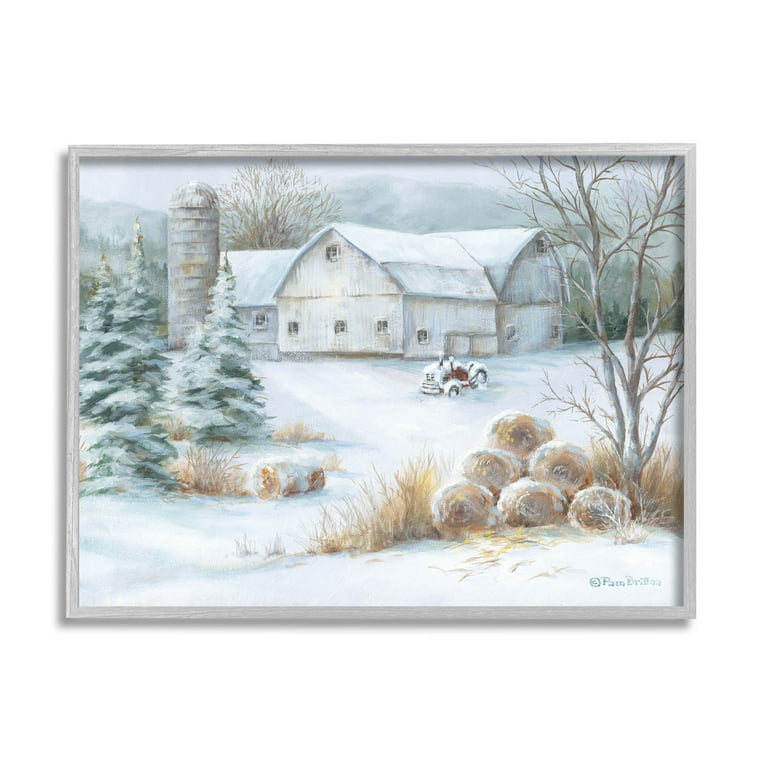A beautifully framed painting, likely a watercolor, depicts a serene winter farm scene. Encased in a wood frame, this artwork features a snow-covered barn and a small silo, set against a backdrop of distant mountains. The scene is enveloped in muted tones of greens, browns, and tans, accentuating the stark, vibrant red of a tractor partially buried in snow, which serves as the painting's focal point. On the left, pine trees, heavy with snow, stand tall next to dried grass and patches of hay. To the right, a leafless tree adds to the wintry atmosphere. In front of the barn, remnants of fallen snow cover the ground, with a copyright mark, possibly attributed to Pam Brilica, subtly visible at the bottom right. The entire painting captures a tranquil and muted winter landscape, highlighting both the beauty and harshness of the season.